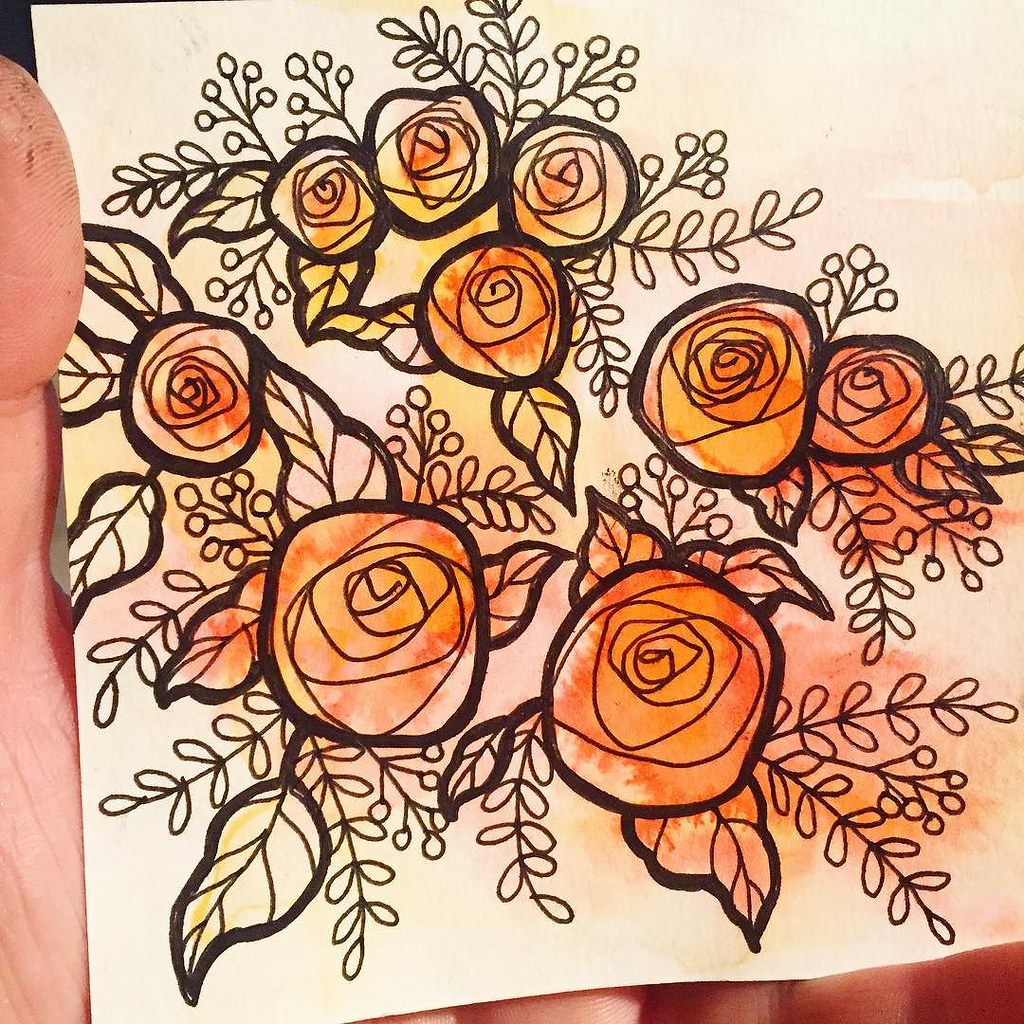The photo is a square, colored image showing a human hand holding up a delicate drawing on what appears to be a cream-colored square piece of paper. The drawing, done in an Art Nouveau style, features a rosebush with nine intricately detailed roses and delicate leaves. The composition includes two orange-red roses at the bottom and additional roses and buds throughout. The roses and leaves are outlined with bold black lines, with finer lines detailing the flowers' interiors. The coloring of the roses is a mix of peachy hues, dabbed on rather than neatly filled in, and a watercolor wash in warm shades of dark orange to yellow fills the background. The drawing is held against the palm of the hand with the thumb visible at the top left, exhibiting some dirt and marks, and the pinky finger seen at the bottom edge, giving a human touch to the meticulously crafted artwork.